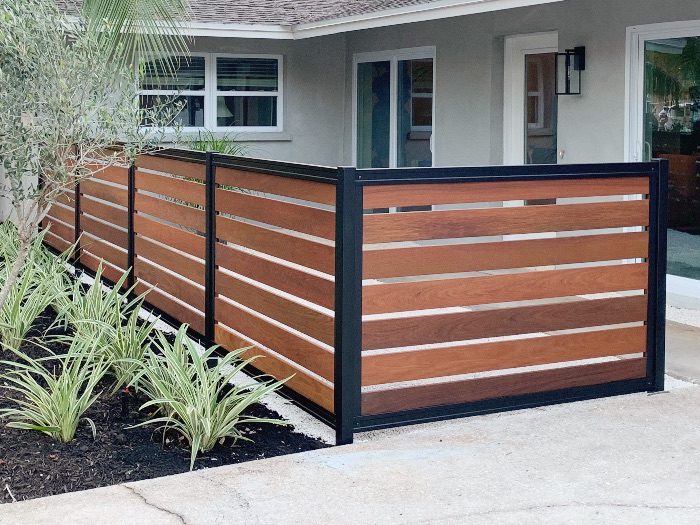This image depicts the backyard of a one-story, light gray ranch-style home. The area features a large square cement patio bordered by a modern L-shaped privacy fence. The fence has a sturdy black metal frame and is filled with seven dark wood planks per panel, each spaced about an inch to an inch and a half apart, allowing for some visibility. On the right side near the corner of the house, there are double sliding doors and a separate door, all with white frames. The backyard also includes a flower bed filled with mulch containing small green plants and a young tree. Scattered around the area are some lighter green plants, contributing to the overall earthy palette comprised of gray, black, brown, and green tones.